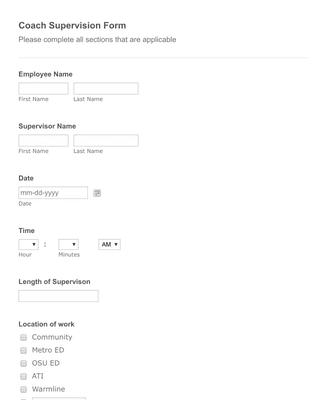**Screenshot Description: Coach Supervision Form Webpage**

The image is a screenshot of a login or registration page on a website, likely intended for registering for an application related to coach supervision. 

At the top, in bold black text, it reads "Coach Supervision Form." Directly beneath this, in standard black text, there is an instruction, "Please complete all sections that are applicable," followed by a thin gray line. 

The first section, labeled "Employee Name" in bold black text, contains two rectangular input fields side by side. The left rectangle is labeled "First Name" below it, and the right rectangle is labeled "Last Name."

The next section, titled "Supervisor Name" in bold black text, similarly contains two rectangles for input, labeled "First Name" and "Last Name."

Following this is a section for the "Date," labeled in bold black text. There is a rectangular input field here marked with "mm-dd-yyyy," accompanied by a small calendar icon to the right. Below the input field, in gray text, it reiterates "Date."

The subsequent section is for "Time," indicated in bold black text. It comprises three small rectangular input fields. The first, with a drop-down arrow, is labeled "Hour" in gray text; the second, similarly styled, is labeled "Minutes;" and the third is labeled "AM" in bold black text, also featuring a drop-down arrow for time selection.

Further down is the section labeled "Length of Supervision" in bold black text. It contains a blank rectangular input field bordered by a gray outline.

The final section, "Location of Work," is marked in bold black text and consists of several dark gray squares, each bearing different labels. The visible squares read "Community," "Metro ED" (with 'ED' capitalized), "OSU ED" (with 'OSU' and 'ED' capitalized), "ATI" (fully capitalized), and "Warm Line" (spelled out as 'W-A-R-M-L-I-N-E').

Overall, the form is neatly organized into clear sections for efficient data entry, featuring both labeled input fields and instructional text for user guidance.